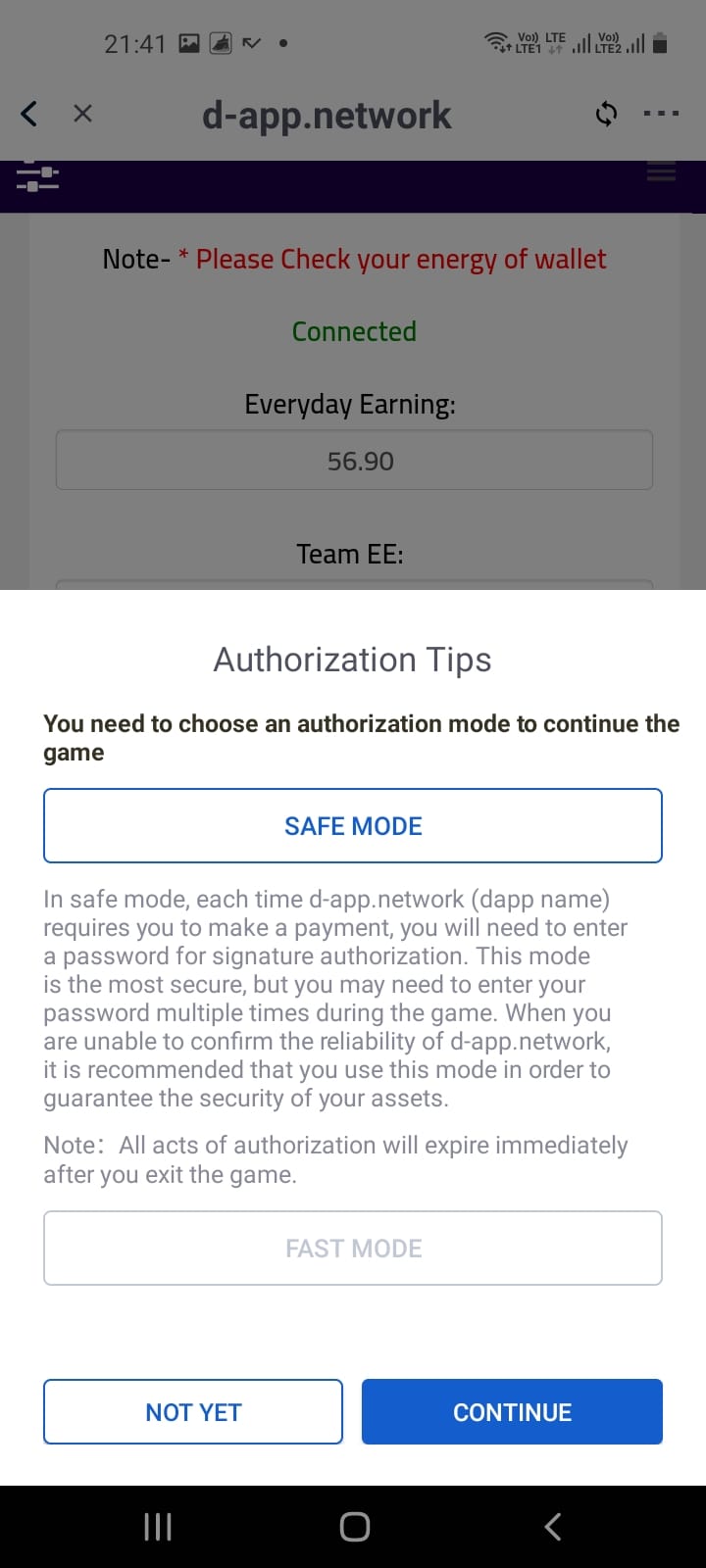The image depicts a portable device screen displaying the "dapp.network" interface. At the top, there are icons indicating Wi-Fi signal strength and battery status. Just below the "dapp.network" header, a shaded box contains a note: "Please check your wallet's energy connected everyday. Earning: $56.90. Team: EE."

Beneath this section, the screen transitions to a white area filled with detailed instructions and information. It starts with "Authorization Tips" and explains the necessity to select an authorization mode to proceed. The "Game Safe Mode" description follows, emphasizing that every time dapp.network requires a payment, users must enter a password for signature authorization. This mode, although secure, may require multiple password entries throughout the game. The instructions strongly recommend using this mode to ensure asset security, especially when the reliability of dapp.network is uncertain. It is noted that all authorizations expire upon exiting the game.

Additionally, there is an option for "Fast Mode" highlighted as a clickable tab. At the bottom of the screen, two tabs labeled "Not Yet" and "Continue" provide navigation options.